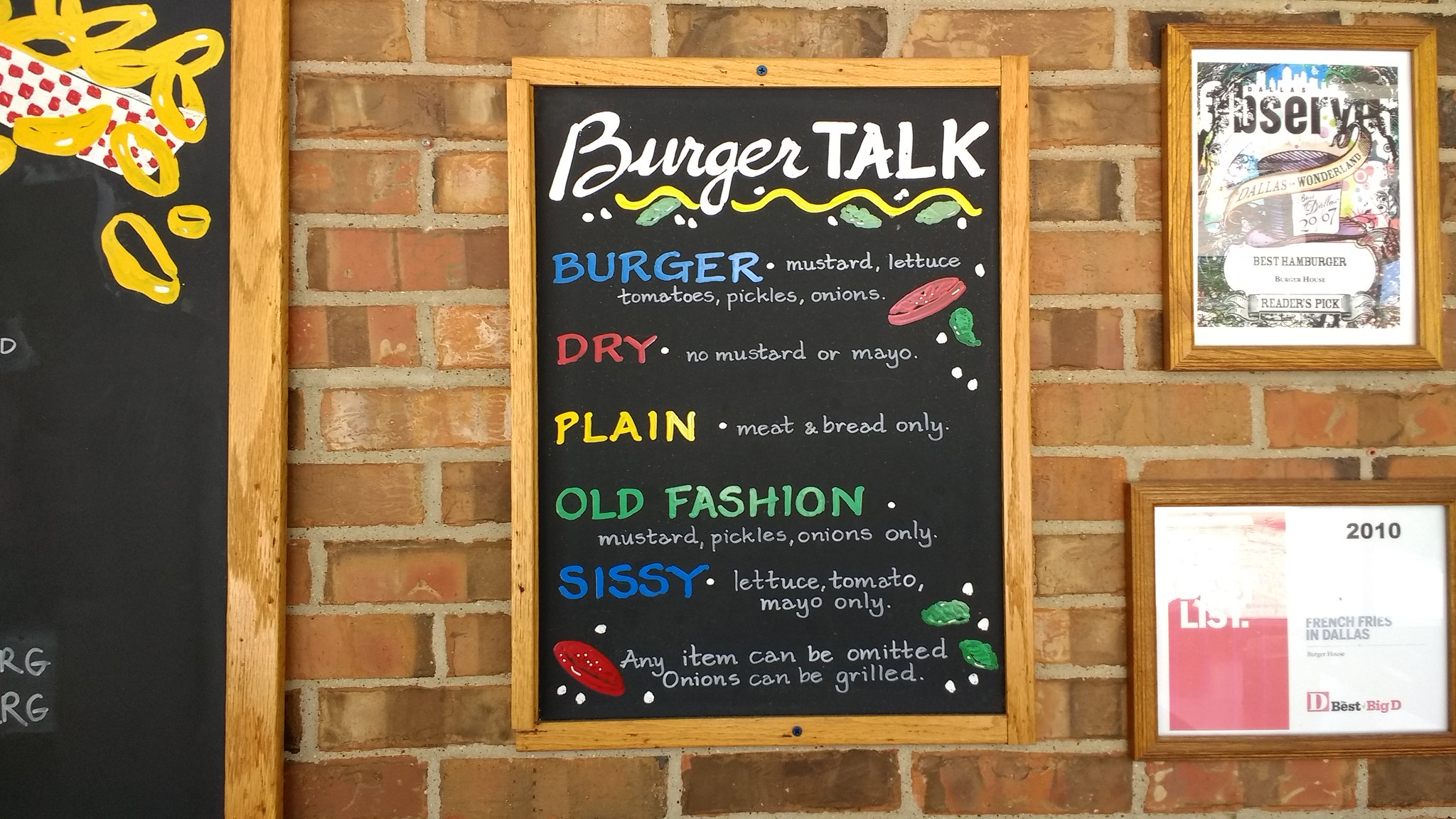The image is a horizontally oriented, close-up color photograph featuring a brick wall inside a restaurant. Mounted on the wall are several framed signs and illustrations. Dominating the center of the image is a chalkboard with a wooden frame. At the top of the chalkboard, the words "Burger Talk" are prominently displayed, with a decorative pattern of leaves and squiggles beneath it. Listed below are various burger options: "Burger," "Dry," "Plain," "Old Fashioned," and "Sissy," each accompanied by a detailed description of its ingredients. The chalkboard is vibrantly detailed in black, white, yellow, green, blue, red, and white colors.

To the left edge of the image, partially cropped off, is a similar chalkboard with an illustrated basket of onion rings featuring red, white, and yellow hues at its upper corner. On the right side of the central chalkboard are two more framed illustrations. The top illustration, enclosed in a wooden frame, depicts a building and appears to be an advertisement. Below it, there is what appears to be a restaurant certificate dated 2010, framed in brown. The certificate is also white, adding a formal touch to the display. The composed arrangement of signs and illustrations provides both informational and decorative elements to the restaurant's ambiance.